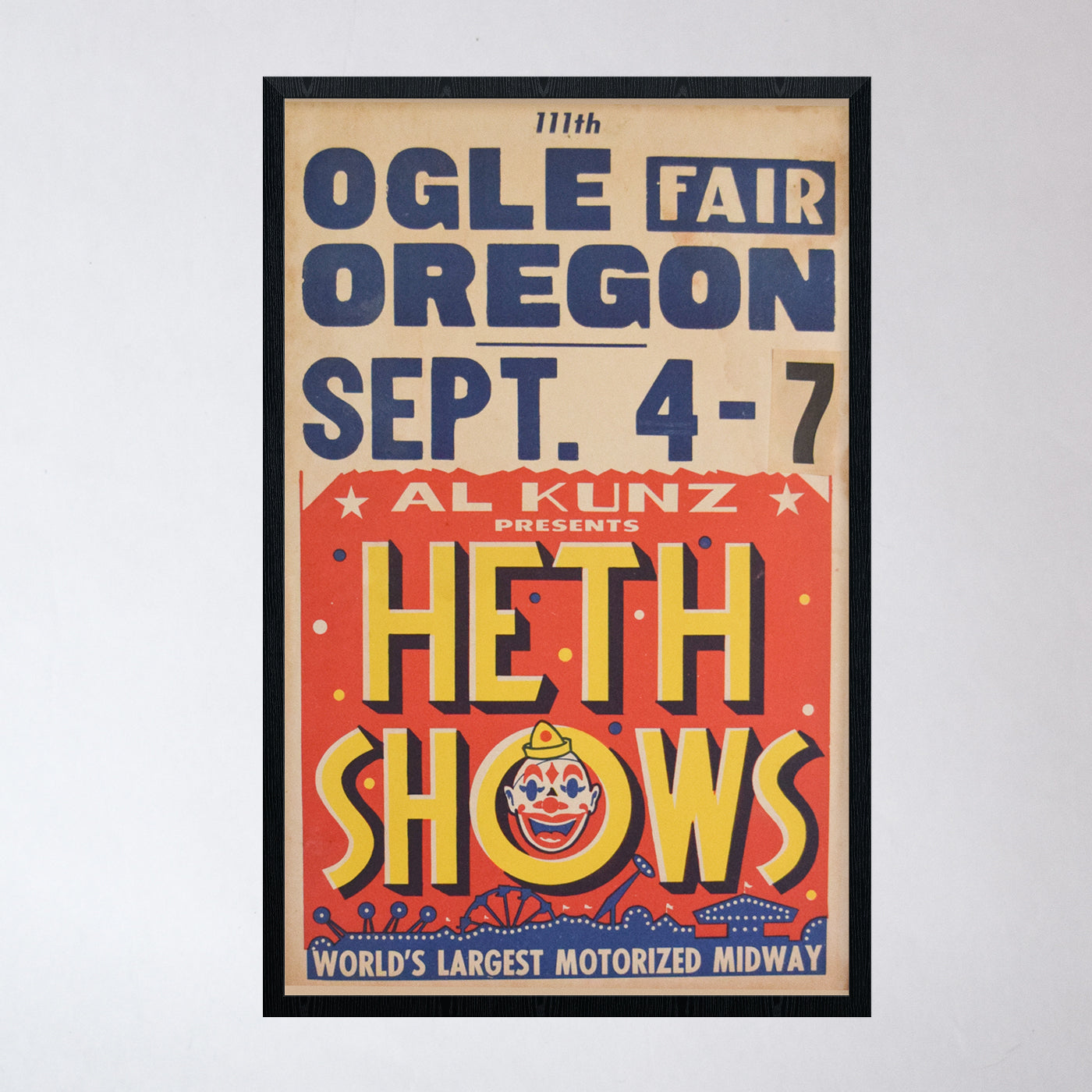This image depicts a framed vintage poster advertising the 111th Ogle Fair in Oregon, taking place from September 4th through 7th (no year specified). The poster, showing signs of aging with stains and a yellowed background, is enclosed in a simple black frame and is set against a white to off-white wall. At the top of the poster, white lettering reads "Al Coons Presents." Below that, in large yellowish-orange letters, it enthusiastically announces "Heath Shows," with the 'O' in 'Shows' creatively featuring a smiling clown face wearing a pointed hat. The lower section of the poster features a vibrant, colorful illustration of the world's largest motorized midway, with circus rides, festive buildings, and lights, resembling a lively carnival scene. The combination of these vivid details and the playful artwork captures the nostalgic charm of a timeless fair.